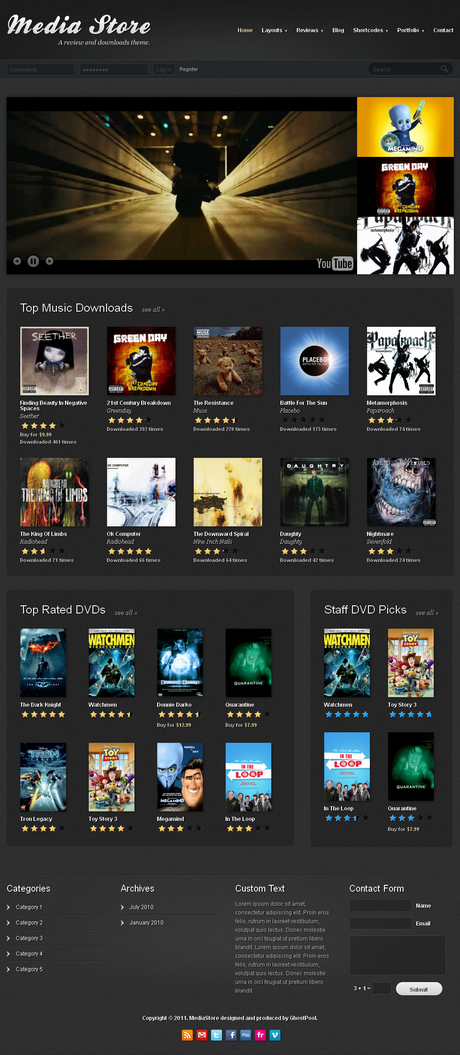The image shows a smartphone screen displaying a variety of digital content available for download. At the top of the screen, there's a section labeled "Tap Music Downloads," featuring numerous square thumbnails with images representing different music selections. Each thumbnail includes the title of the music, the format, a star rating based on user reviews, and the number of downloads it has received.

Additionally, there's a prominent YouTube video visible; it features a nighttime scene of a motorcycle riding up a ramp surrounded by lights. Adjacent to this video, there are three smaller thumbnails for other music videos.

Below this, the screen is segmented into various functional areas including categories for different types of content, archives for previously downloaded items, options for custom text, and a contact form for user inquiries or support.